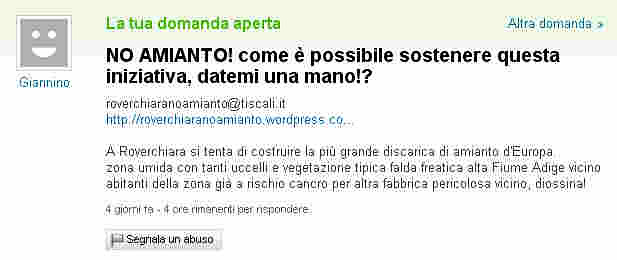The image depicts a social media post, possibly from a website or an ad, written in a foreign language. At the top, in green, it reads "Latua Damanda Aperta L.A. 2 U.A.A D.O.M.A.N.D.A A.P.E.R.T.A." A user named "Giannino," indicated by a gray square avatar with a smiley face, has written the post. Bold black text below the header emphasizes "No Amianto!" with an exclamation point. The post includes an email address and a WordPress link in blue. Additionally, there's a small paragraph in black text and a gray button at the bottom, suggestive of an interaction feature, such as a like or reply button.